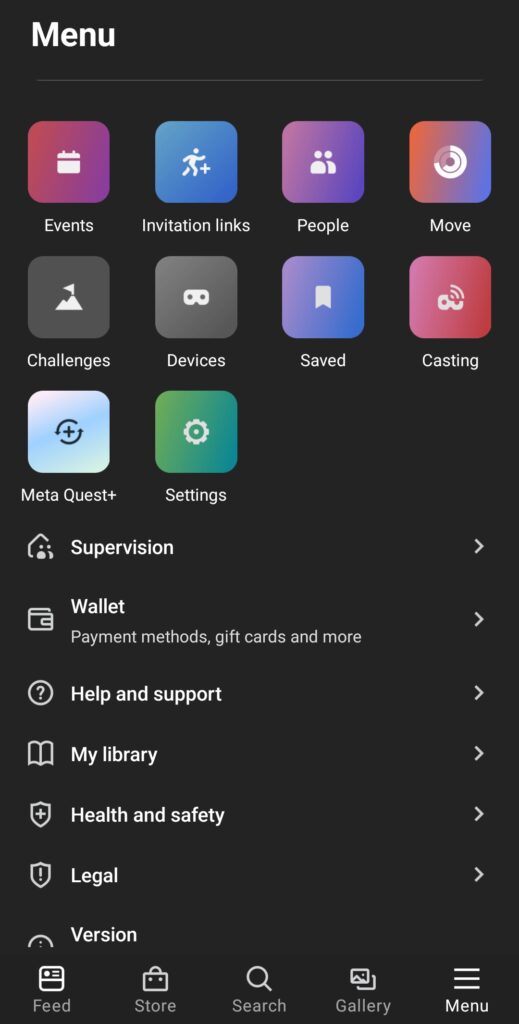In this image, we see a screenshot set against a solid black background. At the upper left corner, in bold white text, is the word "Menu." The first row below this title features a series of square icons, each representing different categories: "Events," "Invitation Links," "People," and "Move." The second row consists of icons labeled "Challenges," "Devices," "Saved," and "Casting." Moving further down, the third row includes "Meta Quest Plus" and "Settings."

Below these rows, the next section presents labeled options in white text: "Supervision" accompanied by an arrow pointing to the right, "Wallet" with a white wallet icon, "Payment Methods," "Gift Cards and More." Further down, there is "Help and Support" represented by a circle with a question mark inside, "My Library" with a book icon, "Health and Safety," "Legal" depicted with an outline of a shield containing a question mark, and finally, "Version."

At the very bottom of the screenshot, spanning from left to right, are five icons labeled: "Feed," "Store," "Search," "Gallery," and "Menu."